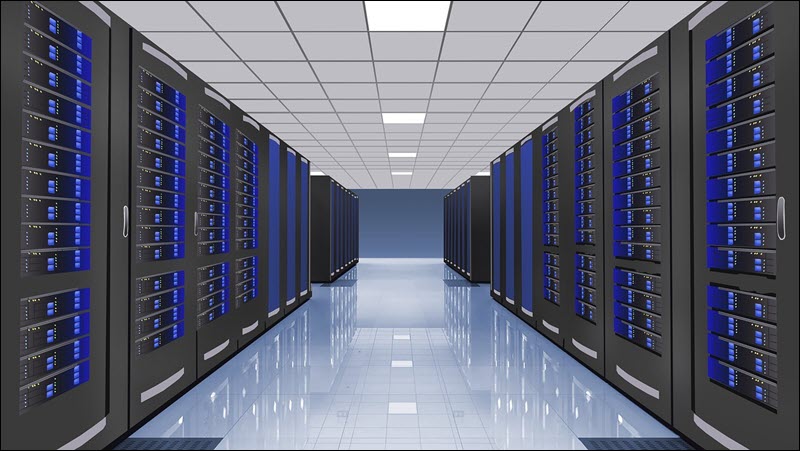The image depicts a detailed, computer-generated rendering of a large, high-tech server room or data center. The corridor runs deep into the building, bordered by sleek, oblong black cabinets filled with rows of blinking blue lights and numerous computer components, each cabinet framed with silver strips and handles. The polished white tile floor reflects the bright, fluorescent lighting from the drop tile ceiling, which consistently features lights embedded every few tiles. The scene lacks windows, enhancing the clinical, purpose-driven ambiance typical of basements or secure, windowless IT infrastructure spaces. Toward the far end of the hallway, a slate blue wall can be glimpsed, adding a touch of color contrast to the mostly monochromatic and metallic environment.